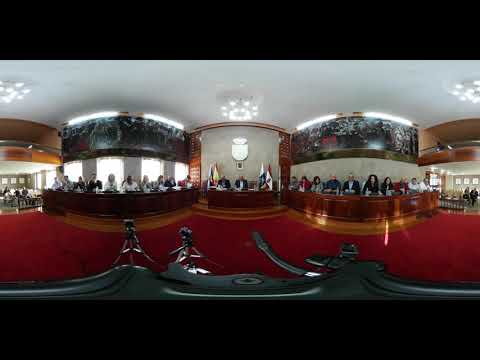The image depicts an indoor scene of what appears to be a press conference, legislative assembly, or a formal meeting. The room features a red carpeted floor contrasted by a white ceiling, which is illuminated by several chandeliers and ceiling lights that add a warm glow. At the front of the room, there is a long, white desk with two people seated behind it, flanked by four small flags that are difficult to identify. The seating arrangement is sectional, with curved wooden benches on both the left and right sides, each accommodating around ten middle-aged individuals dressed in business attire, including suits, jackets, and blazers. Additional people are visible along the far left and right edges of the room, with some still entering through open doors located at the far ends. The image is slightly distorted, reminiscent of a fisheye or surveillance camera perspective. In front of the seating area, there are cameras and additional lighting set up, indicating that the event is being recorded or broadcast. The overall ambiance suggests a formal, governmental or international context, marked by the presence of multiple national flags and the business-like demeanor of the attendees.